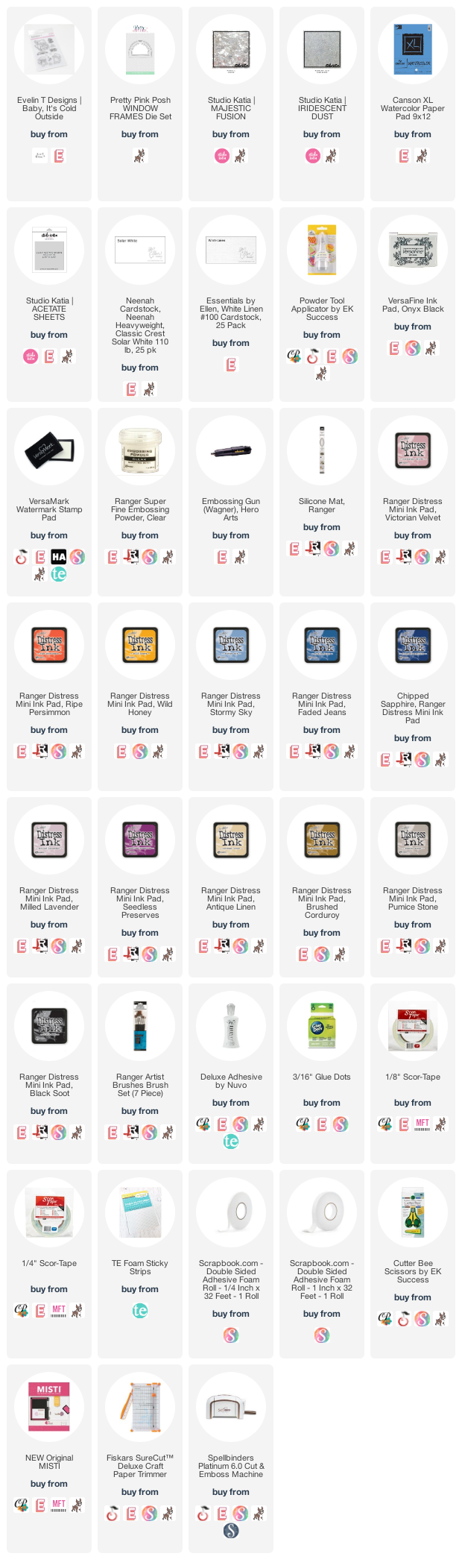The image appears to be a digital grid or table with a total of 38 squares, organized into rows of five. Each square features a gray background with a white circle or oval at the top, followed by an image of an item inside the square. Below each item, there is a short description and a series of icons, varying in number from one to six or more. Some of these icons are discernible, including a briefcase, a smartphone cover, and a spatula, among others. The overall appearance is somewhat blurred and unclear, making the specific details and text difficult to read.